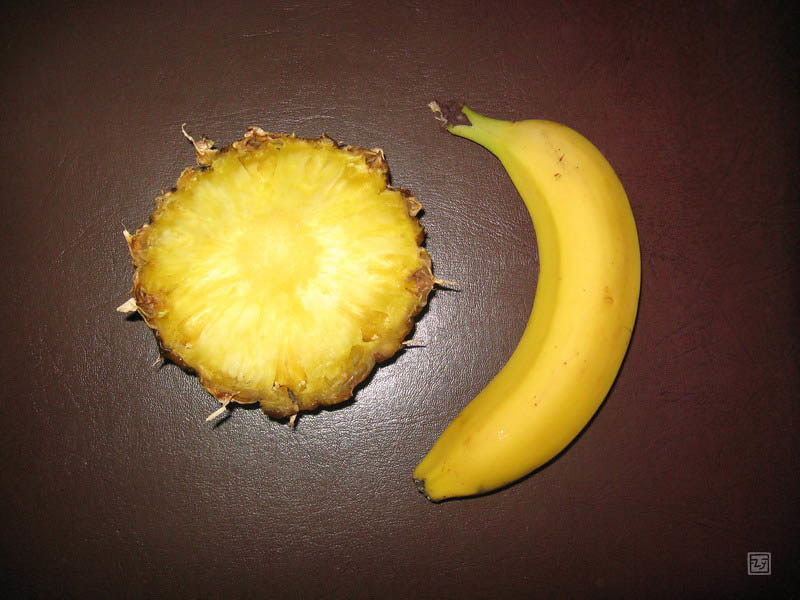The image captures a selection of fruit placed on a brown table or counter. In the bottom right corner, there is a white watermark depicting a simplistic face with two small dots for eyes, an L-shaped nose, and a curved line for a mouth, all within a square outline. The background of the image shows a painted surface with visible ridges and lines. The edges of the image, especially the top right, top left, bottom left, and bottom right corners, appear darker. 

At the center of the image, there is a round slice of pineapple with the exterior skin still attached, showing a slightly fuzzy texture. The pineapple slice has a dehydrated appearance, with a yellow center indicating it has been left to dry out. Beside the pineapple slice is a whole banana with a greenish stem, a yellow peel, and a few brown and black spots, suggesting it is ripening.